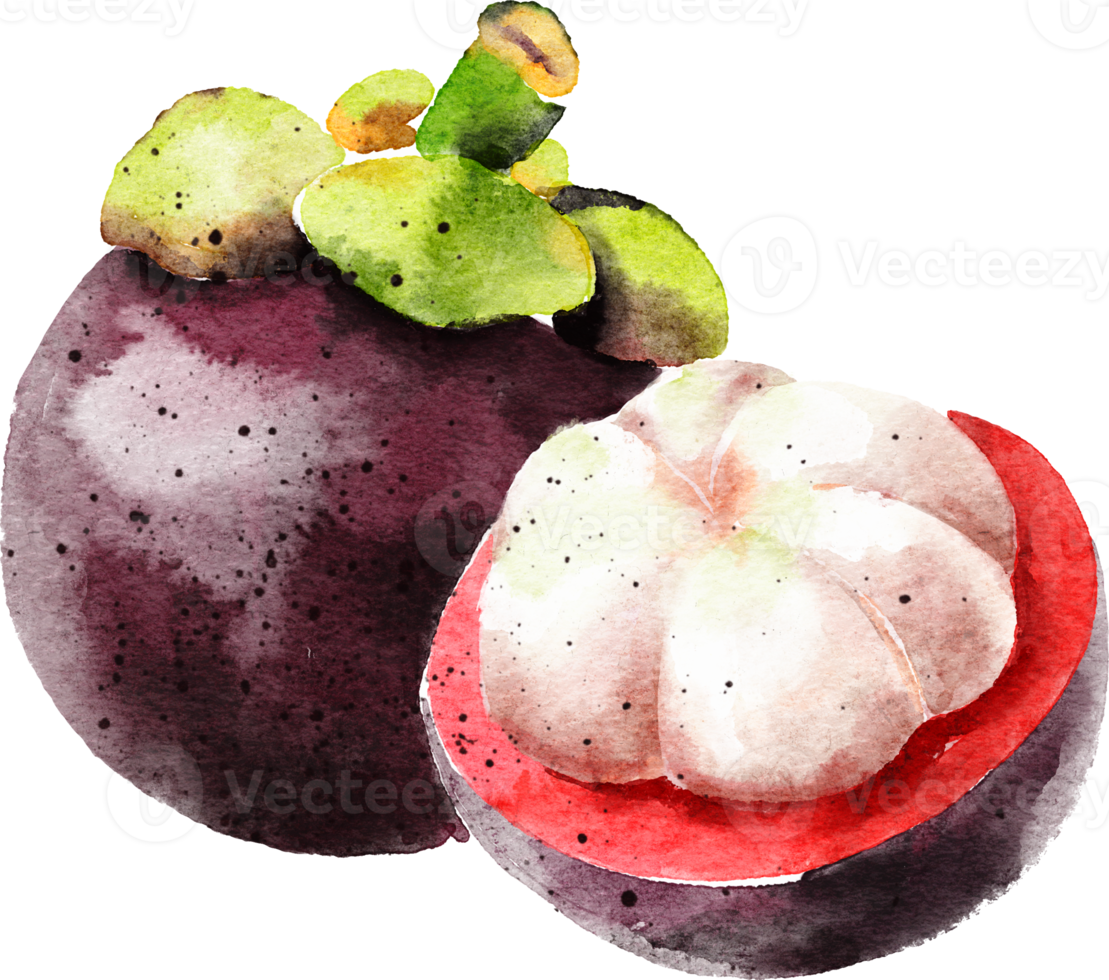The image depicts a watercolor painting of a round, dark purple fruit with a multitude of black specks scattered across its surface. On the left side of the image, there is a whole version of this fruit, crowned with thick, chunky green leaves surrounding its stem, which exhibit some black-tinged edges. The fruit has a grape-like appearance, with subtle lighter sparks adding depth to its hue. On the right side, a halved version of this fruit showcases a richly red interior rim, contrasting sharply with a central white section that is somewhat rounded and textured, bearing a resemblance to a mushroom cap or part of a garlic clove. This white section adds an intriguing element to the composition, with delicate yellow tones at its center. The detailed portrayal captures the texture and color intricacies with a gentle light shine highlighting the features. Additionally, the bottom of the image carries a faint watermark that reads "V-A-C-T-E-E" or something similar.